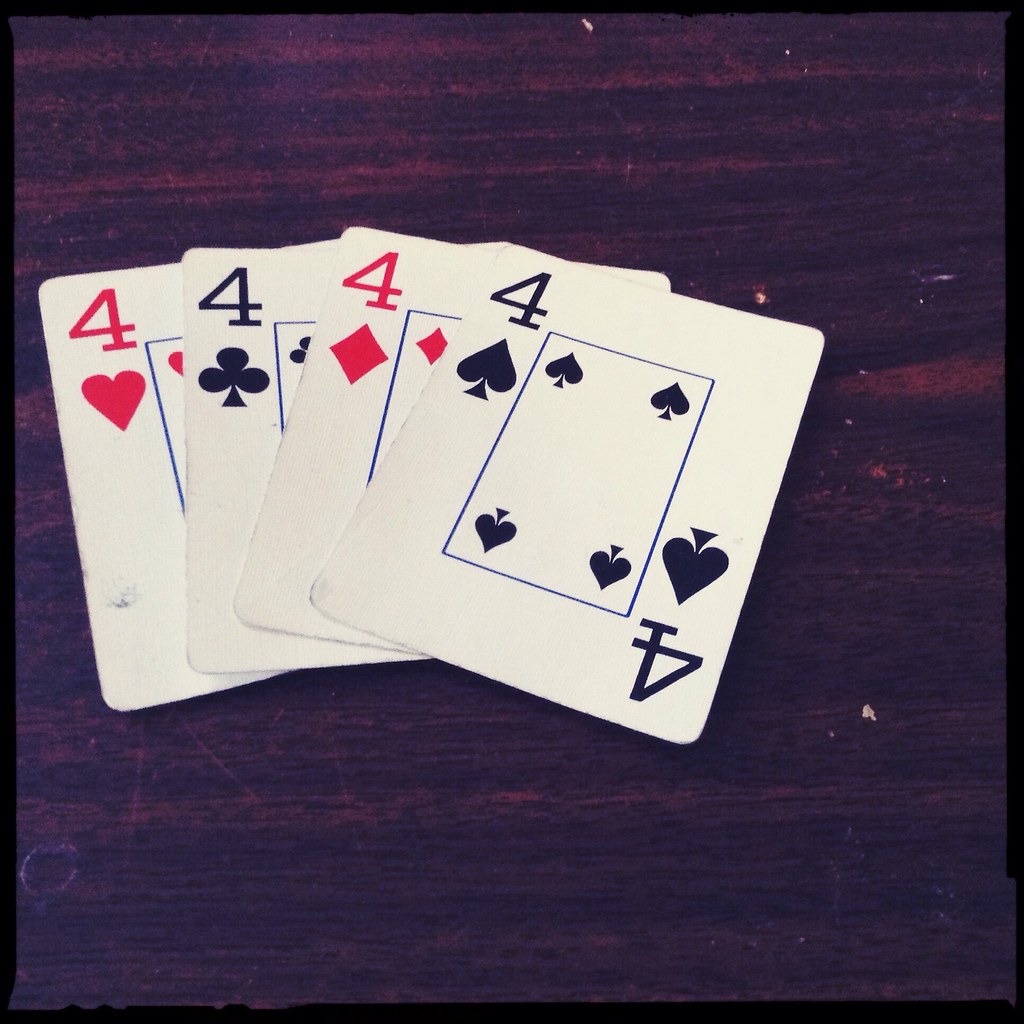A close-up photograph showcases four playing cards meticulously arranged on a dark wooden surface. Only the top-left corners of the cards are visible, revealing their suit and rank. From left to right, the cards are four of hearts, four of clubs, four of diamonds, and four of spades. Each card features a distinctive design: a blue square encloses four miniature symbols that correspond to the card's suit. For example, the four of spades has four small spades within the blue square, along with an additional spade beneath the digit "4" in the top left and a mirrored spade in the bottom right corner. The back of one card is visible, providing a clear view of the design and confirming the configuration of the other three cards. The dark wood background enhances the contrast and detail of the cards, making the intricate designs stand out prominently.